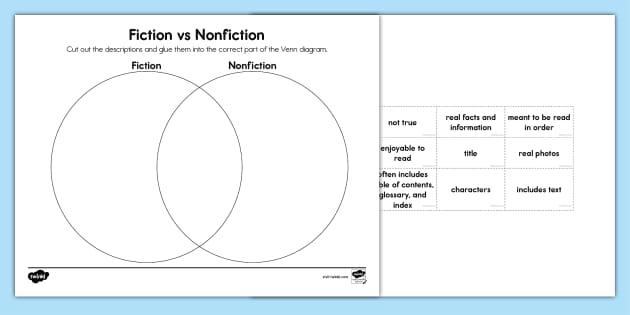The poster appears to be a teaching aid for either a journalism or literature class, titled "Fiction Versus Nonfiction." It features a clean white background with black lettering, encased in a blue frame. On the left side of the poster, the title "Fiction Versus Nonfiction" is prominently displayed. Below the title is a Venn diagram with two overlapping circles, one labeled "Fiction" and the other labeled "Nonfiction." The central overlapping area is reserved for characteristics common to both genres. On the right side of the frame are individual descriptors meant to be cut out and placed in the appropriate sections of the Venn diagram. These descriptors will help differentiate and identify attributes specific to fiction, nonfiction, and those shared by both.